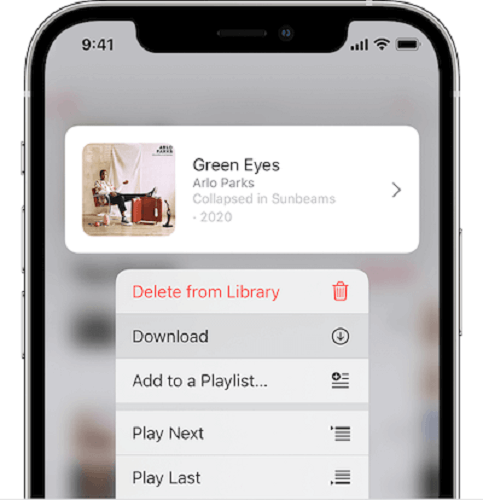A detailed view of a smartphone screen displaying the Apple Music interface. The device shows the time as 9:41, with a full battery, Wi-Fi connection, and maximum signal strength. Centrally, the screen presents the song "Green Eyes" in bold black text, followed by the artist's name, Arlo Parks, in lighter print. The album title "Collapsed in Sunbeams," and its release year, 2020, are listed below the artist's name. A picture of Arlo Parks is visible, featuring them seated on wooden furniture with a white curtain behind, adding a personal touch.

To the right of the album details, a black arrow invites users to access more information. Below this section, options include a "Delete from Library" command in red, accompanied by a red trash can icon. Another selectable option, "Download," is highlighted in black with a circle-enclosed arrow icon. Additional actions are available, including "Add to a Playlist" with an arrow and lines icon, "Play Next" with a single arrow and lines icon, and "Play Last" with a similar configuration.

Each element on the screen is clearly delineated, providing a robust set of choices for managing and enjoying the musical content.